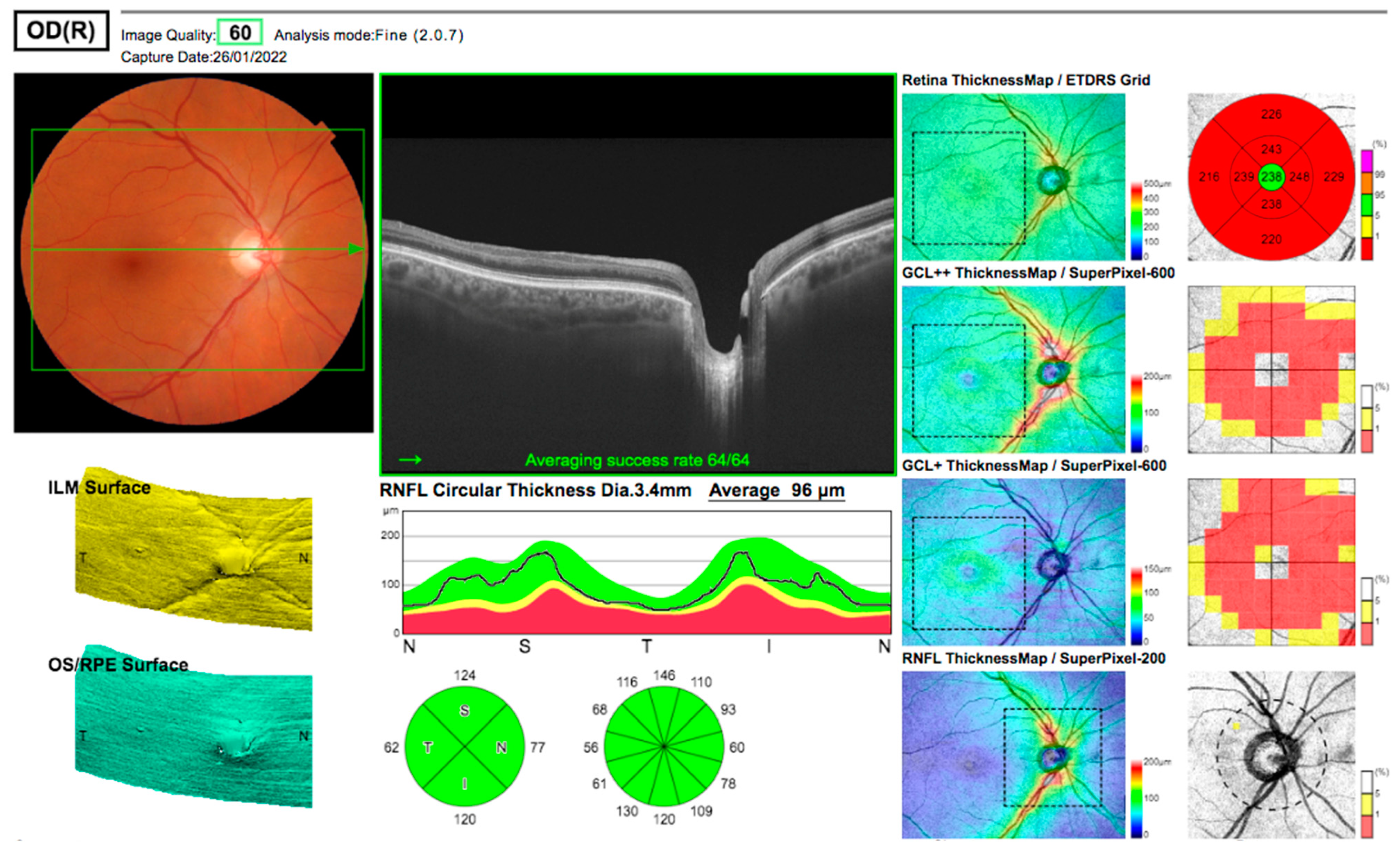This is a detailed, horizontal color infographic displaying various components and measurements related to an eyeball. In the top portion, a rectangular section features the text "OD (R)" with "Image quality: 60" in smaller black font to the side, enclosed in a turquoise rectangle, and "Analysis mode: find (2.007)" beside it. Below this header, the capture date "26/01/2022" is noted.

Dominating the left side is a series of illustrations and charts focusing on the eye. At the top right, there's a vivid image resembling an eyeball with a bright orange circular shape marked by thin red lines, resembling veins. Below this, there's a dark rectangular image that appears to depict terrain with different land features and a labeled "Average success rate: 64/64."

The middle section includes text labels like "ILM surface" with yellow areas and "OS/RPE surface" shown in green. An averaged success rate image is tagged with dimensions and further information. To the right, multiple smaller images display green and blue terrain-like maps and retina thickness details. Highlighting specific measurements, the diagrams list "RNFL circular thickness" with a specific diameter of "3.4 mm" and an average measurement of "96 new mm."

On the far right, eight various charts detail "Retina thickness maps," "GCL+ thickness map," and "RNFL thickness map." Additionally, two green pie charts at the bottom provide segmented data with sections labeled numerically.

Interconnecting black lines that resemble branches run throughout the diagram, linking various images and charts. A turquoise rectangle and an adjacent yellow rectangle are also present on the left side. Below these, a fluctuating graph depicts mountain-like peaks and valleys in green, yellow, and red hues, indicating different measurements or values.

Overall, this intricate medical diagram comprehensively details different attributes and measurements of the eye, incorporating multiple charts and visual elements to convey diverse data points.